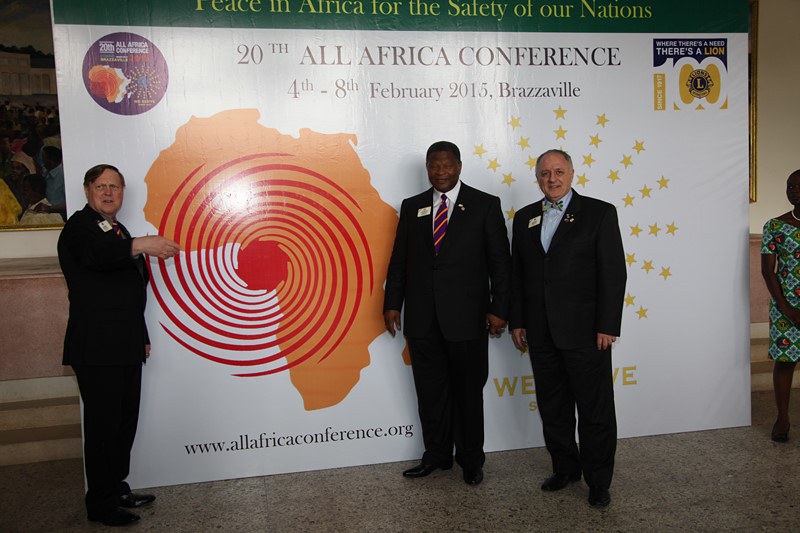In this photograph, three men stand in front of a large white banner with dark red text that reads "20th All-Africa Conference, 4th to 8th February 2015, Brazzaville." The banner features additional phrases such as "peace in Africa for the safety of our nations" and "where there's a need there's a lion." The banner also includes an orange map of Africa with a red spiral image, resembling a hurricane, over the west coast of the continent. Flanking the central text, there are two symbols: an orange circular image on the left and a yellow and blue square image on the right. 

In the center, two men in dark suits stand side by side. The man on the left is a black man wearing a tie, while the man on the right is a lighter-skinned man wearing a bow tie. To the left of these men, another individual is captured pointing towards the board, drawing attention to the African continent illustration. Additionally, a black woman in a dress is partially visible on the right edge of the image. The bottom left of the banner includes the text "All Africa Conference dot org."